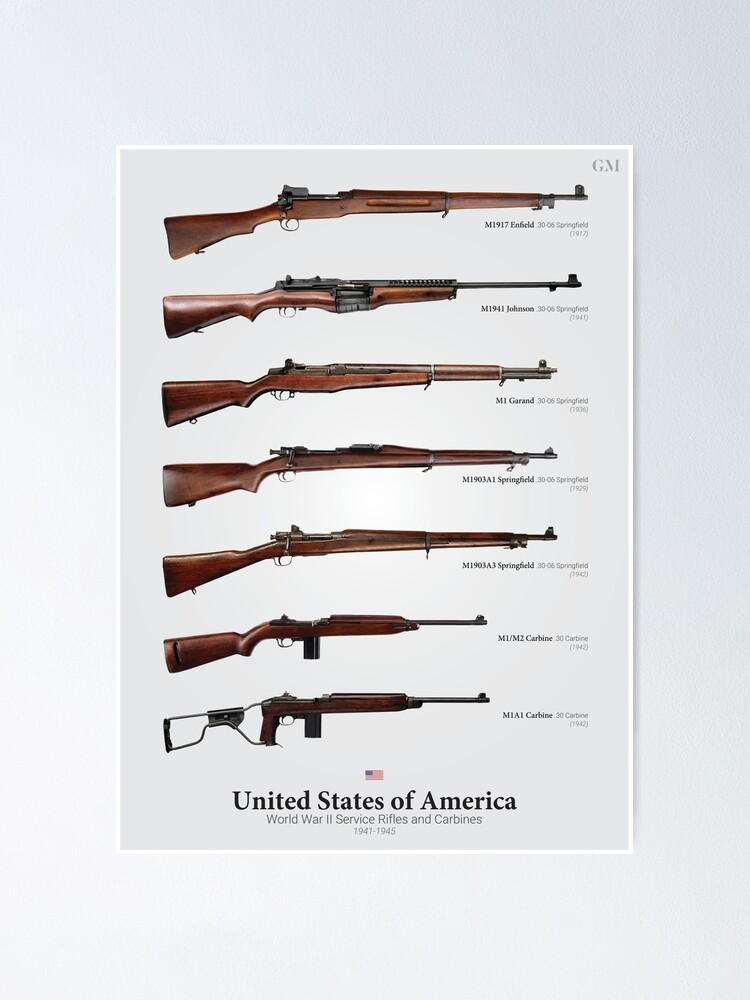This detailed poster features a collection of World War II service rifles and carbines used by the United States from 1941 to 1945, displayed against a slightly grey background. In the foreground, the white poster has a thin border and is centered within this grey backdrop. At the bottom, in black text, it reads "United States of America" with a small American flag above it, followed by the annotation "World War II Service Rifles and Carbines 1941-1945."

The poster is a visual, vertically descending list of seven firearms, each depicted from a side angle with their barrels facing to the right. Each gun is crafted from wood with metal components. The sequence starts with the M1917 Enfield (30-06 Springfield, 1917), a long rifle with a wooden muzzle. This is followed by the M1941 Johnson (30-06 Springfield, 1941), differentiated by its metal top and clip feed. 

Next is the M1 Garand (30-06 Springfield, 1936), notable for its shorter muzzle. This is succeeded by two versions of the Springfield rifle: the M190A1 Springfield (30-06 Springfield, 1929) and the updated M1903A3 Springfield (30-06 Springfield, 1942). 

Following the rifles is the M1/M2 Carbine (30 Carbine, 1942), distinguished by its shorter stock and muzzle along with a bottom-placed clip. The final firearm is the M1A1 Carbine (30 Carbine, 1942), unique for its foldable metal stock, contrasting with the wooden stocks of the other firearms.

Each gun’s name and specifications are labeled directly underneath its barrel, offering a comprehensive view of the evolutionary modifications of these WWII service rifles and carbines.